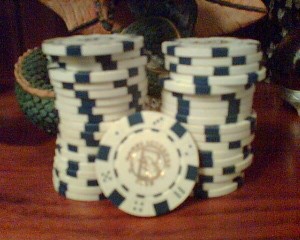In this color photograph, a pair of stacks, each consisting of roughly 20 to 25 poker chips, are prominently displayed on a dark wooden surface. The chips are primarily white with six evenly spaced black sections around the edges, and each chip features a central silver logo. Interspersed among the black sections are various dice dots arranged in numerical patterns, adding intricate details to their design. Between the two stacks, one poker chip stands upright, leaning against the stacks and facing the camera. The background is faintly visible and appears to include a brown and green wicker basket, though it remains somewhat indistinct due to the blurriness of the image. The primary focus remains clearly on the poker chips, with no other significant objects, people, animals, or plants present in the photograph.